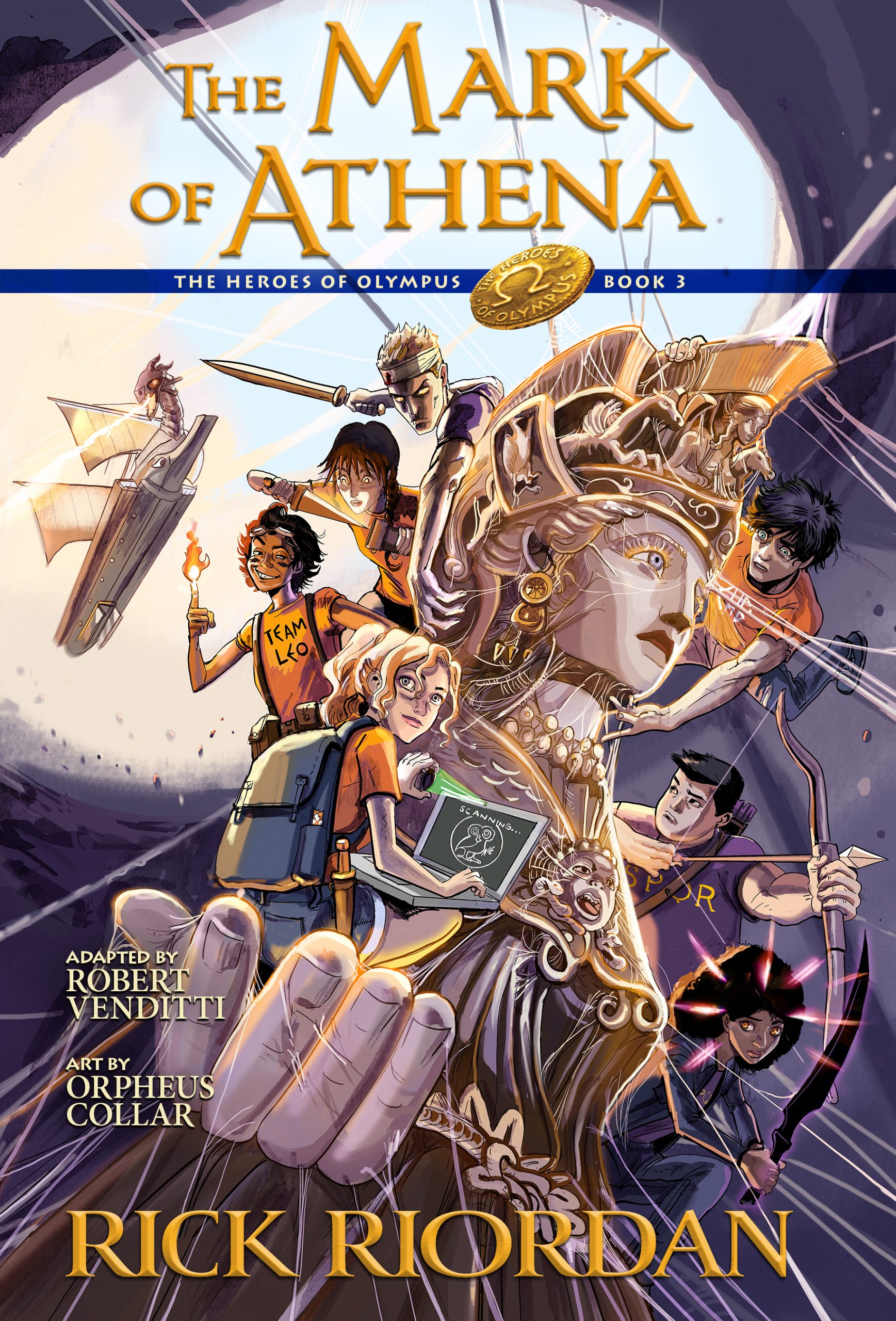This is the cover of the young adult fiction novel "The Mark of Athena" by Rick Riordan, part of the Percy Jackson series. At the very top, in yellow handwriting, it says "The Mark of Athena," beneath which, in white lettering across a blue strip, it says "The Heroes of Olympus, Book 3." The overall illustration style is reminiscent of a blend between anime and American modern comics.

Dominating the cover is a colossal statue of a female warrior, presumably Athena, with an elaborate headpiece. The statue has its hand extended outward, and standing on the hand is one of the characters – a young person holding a bow and arrow. Surrounding the statue are seven kids, each equipped with different weapons and items. On the right side, one character wields a bow, while another holds a sword. On the left side of Athena's bust, another set of kids can be seen: one with a computer, another with a small flame, one with a dagger, and the highest figure holding a sword. A Viking ship, complete with a dragon head and sails, floats through the air in front of a giant, moon-like opening in the background, suggesting they are about to enter a cave.

At the bottom left, it says, "Adapted by Robert Venditti, Art by Orpheus Collar," in white text. In larger gold writing at the very bottom, it is signed "Rick Riordan," indicating the author of the novel. Overall, the background appears to depict a nighttime scene, enhancing the adventurous and mythical atmosphere of the cover.